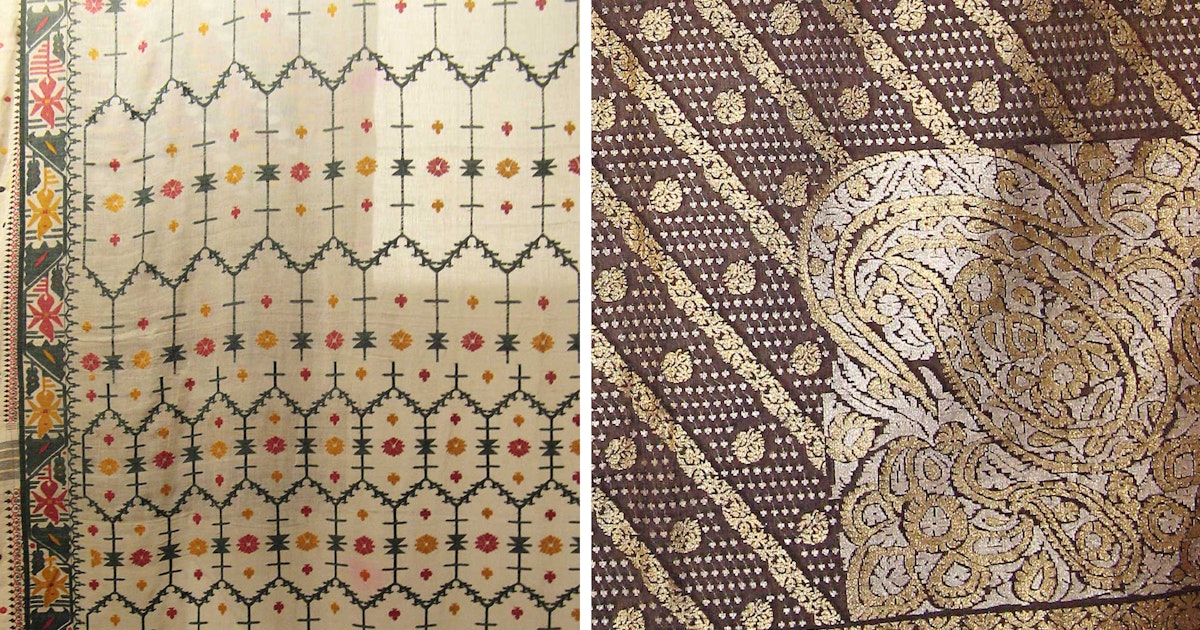The image showcases two pieces of elaborately designed tapestry side by side. The left tapestry, set against a light cream background, features a vibrant array of oblong diamond shapes organized in neat rows. These shapes are filled with intricate, tiny woven flowers in shades of muted red, darker green, and gold. The piece is bordered with deep, contrasting colors, complementing the floral motifs within. The right tapestry is more subdued, exhibiting a chocolate brown background adorned with diagonal gold stripes and sprinkled with white and larger gold dots. In the bottom right corner of this piece, there is a large, ornate paisley-like pattern in golds, blacks, and whites, adding an element of intricate elegance to the overall design.